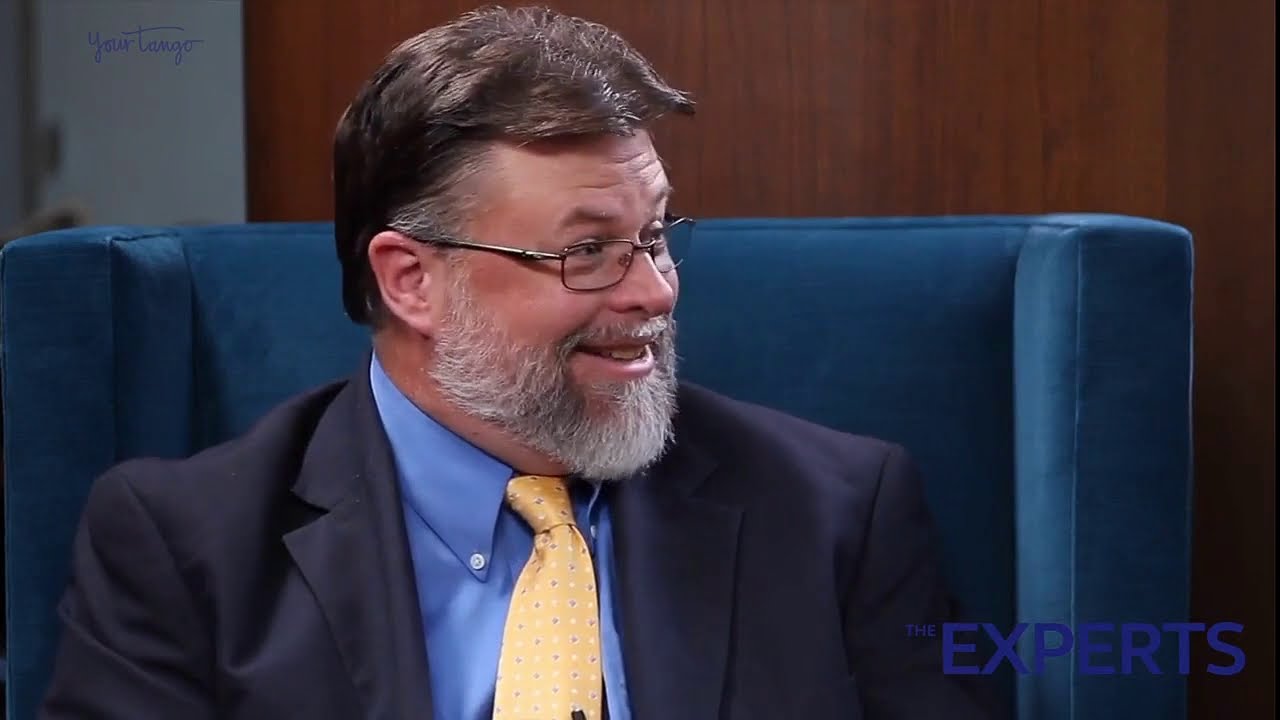The image is a high-resolution photograph showing a man sitting in a large blue chair. The setting features a primarily brown wooden wall backdrop with a small section of white wall in the top left corner, possibly with a door. On the white wall, blue cursive writing spells out "Your Tango." The man is positioned slightly off-center to the left, and the photograph captures him from his chest to the top of his head as he looks to his left. He has brown and gray hair that falls just past his ears, and he sports a gray beard and mustache. He wears glasses and is dressed in a dark blue blazer, a lighter blue button-up shirt, and a yellow polka-dotted tie. He appears to be smiling in a somewhat sarcastic or surprised manner. In the bottom right corner of the image, the text "The Experts" appears in blue font. The color palette of the image includes shades of blue, yellow, brown, tan, black, and gray, and the overall style suggests a formal or debate-type environment.